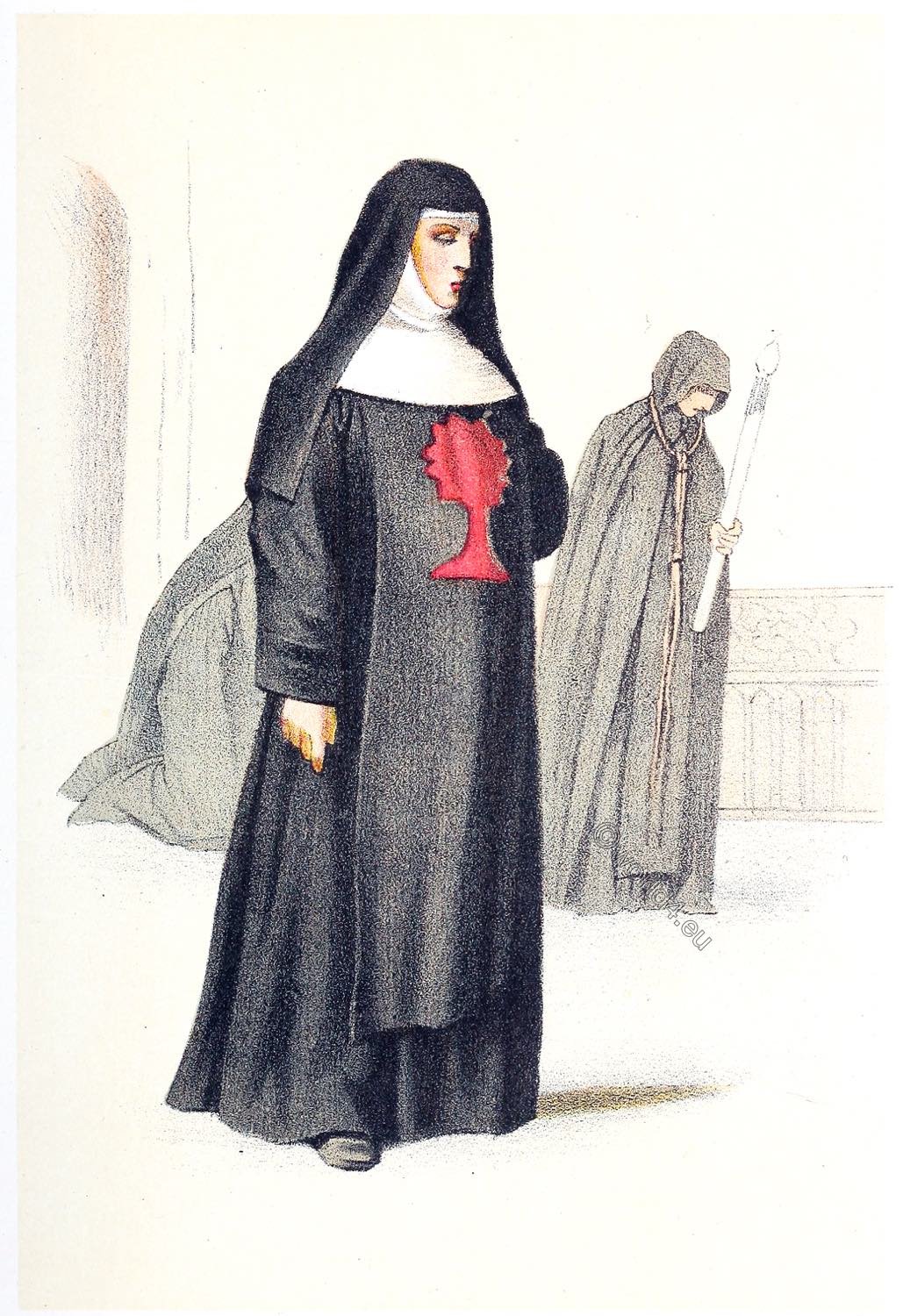The image is a detailed vintage illustration, reminiscent of styles from the 1800s, likely executed with either colored pencil or brush. It portrays a nun in a black habit adorned with a red emblem resembling a sun on a pedestal emblazoned on her chest. Her eyes are gently closed, and she gazes downward with a serene expression. The monochrome background adds to the antique feel, complemented by muted color tones. Behind the nun, two additional robed figures are depicted: one kneeling and partially obscured, visible only by a back leg, while the other stands in the background on the right, holding a tall candle. The overall setting and composition suggest a scene that could be found in an old book, conveying a sense of timeless reverence and tranquility.